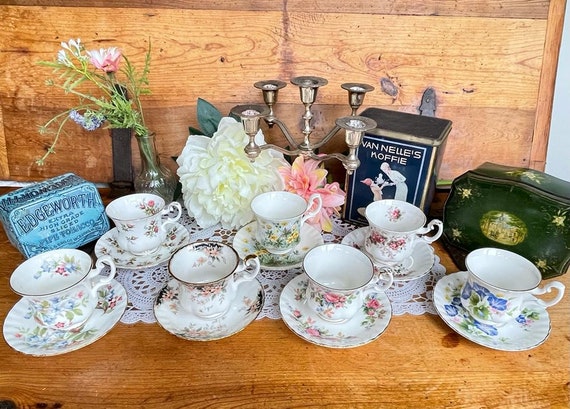This detailed photograph showcases a charming collection of seven vintage teacups, each paired with a matching saucer, arranged on a delicate lacy placemat set atop a light-stained wooden surface. The teacups, displayed in two neat rows—with four in the front and three behind—all feature intricate floral patterns, reflecting an array of colors including blue, pink, yellow, green, and multicolored designs. Each cup boasts an ornate handle on the right side. Beyond the teacups, a quaint assortment of decorative vintage items graces the background: a vase brimming with green stalks and pink and purple flowers, a five-candle candelabra, a rectangular blue case labeled "Edgewood Extra High-Grade Sliced Pipe Tobacco," a metallic box marked "Van Nels Koffie" with an image of two figures, and a green container adorned with white flowers and a central oval design. The setting evokes a sense of nostalgic elegance, highlighted by the warm wooden backdrop.